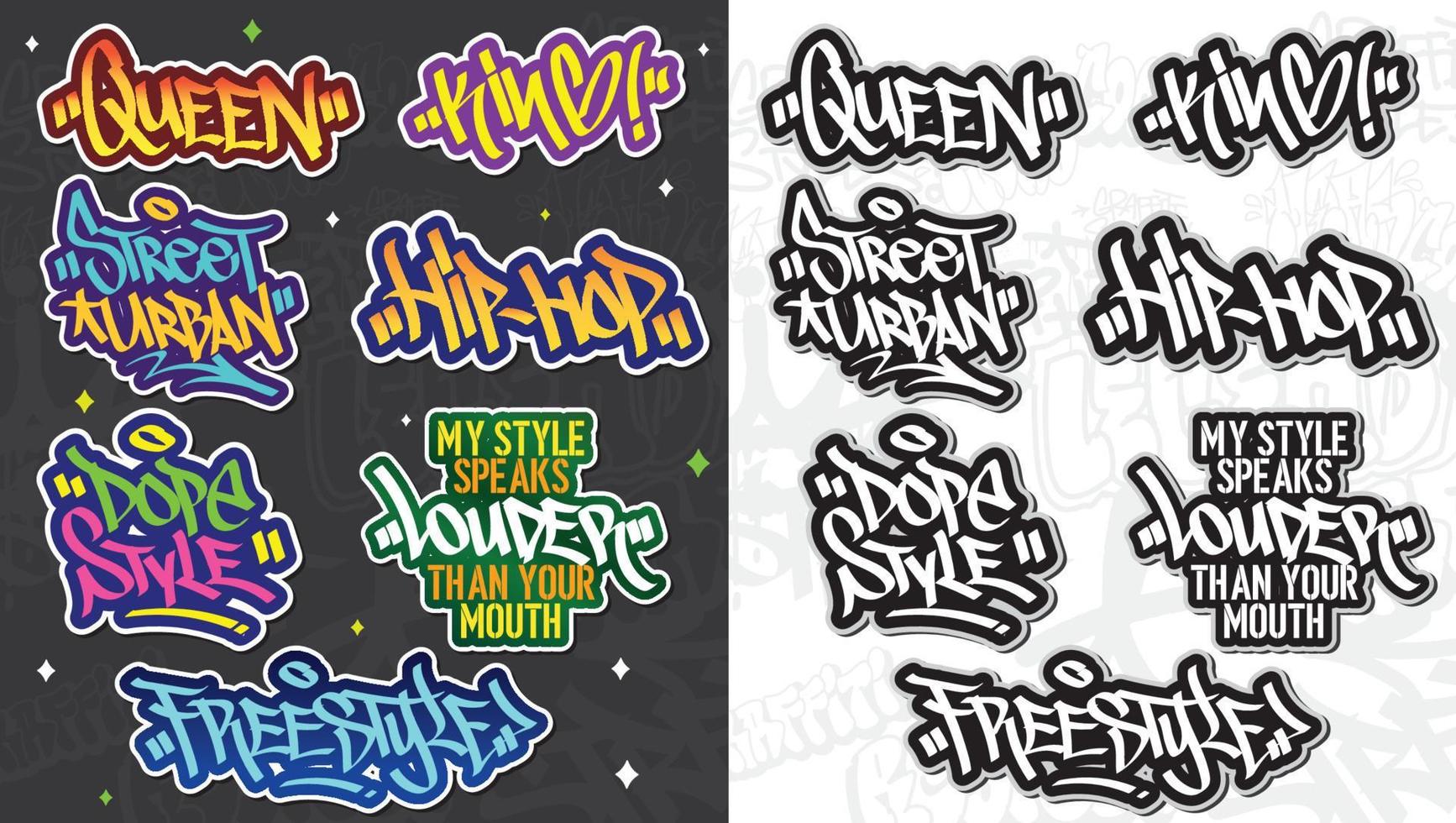The image showcases two posters side by side, displaying the same sequence of graffiti-style text but with distinct color schemes. The left poster features vibrant, multicolored text on a black background. The first line reads "Queen" in an orange and red gradient. Below it, “Street Urban” is written in blue and yellow. The third line, “Dope Style,” displays a mix of green, pink, and yellow. At the bottom, “Freestyle” stands out in light and dark blue shades. The right-hand side poster presents the same words, but in black and white on a white background, providing a stark contrast to the colorful left side. Additionally, the text “Kin” or “Kind” and "Hip-Hop" appear on the left in pink and purple and orange, yellow, and dark blue respectively, while the phrase "My Style Speaks Louder Than Your Mouth" is highlighted in yellow, orange, white, and green on the left. Both posters depict the same statements but emphasize different visual aesthetics — one with vibrant colors and the other in monochrome.